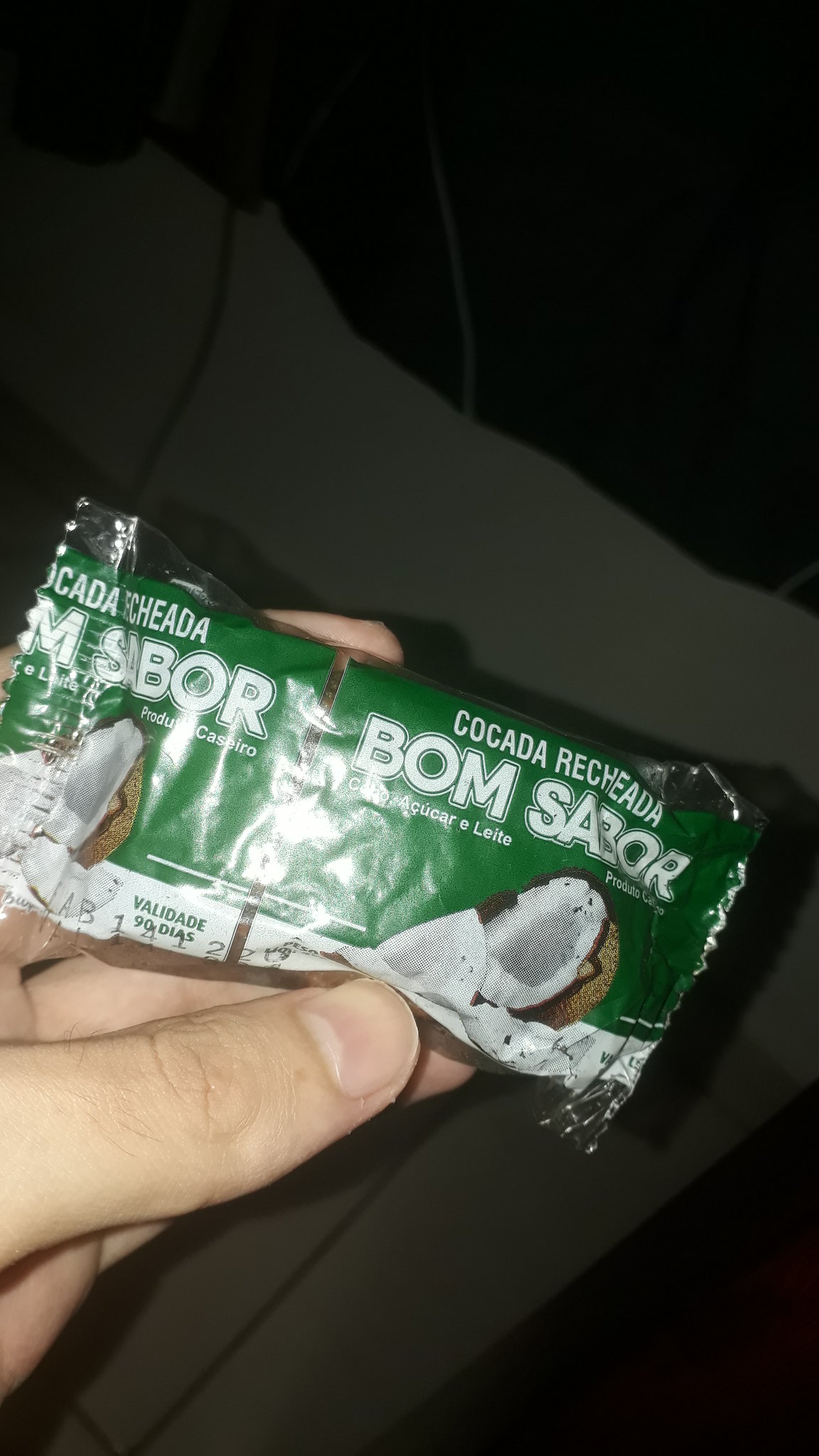The image features a candy bar wrapper being held by a hand emerging from the bottom left of the frame. The setting appears dark, hinting at an indoor environment, possibly with some fabric visible in the background. The hand holding the candy bar, likely belonging to a man, exhibits a clipped thumbnail with the fingertips partially visible above the wrapper. The wrapper itself is predominantly green with a white strip along the bottom and displays the branding "Kolkata Recheada" in smaller white letters at the top, and in larger white letters underneath, "Bom Sabor." Below this, there is smaller text obscured by a glare. A realistic image of chocolate is situated on the bottom right. Additionally, two white boxes are visible, one clearly reading “VALIDADE 90 DIAS” (valid for 90 days), with some barely legible black printed numbers likely indicating an expiration date.